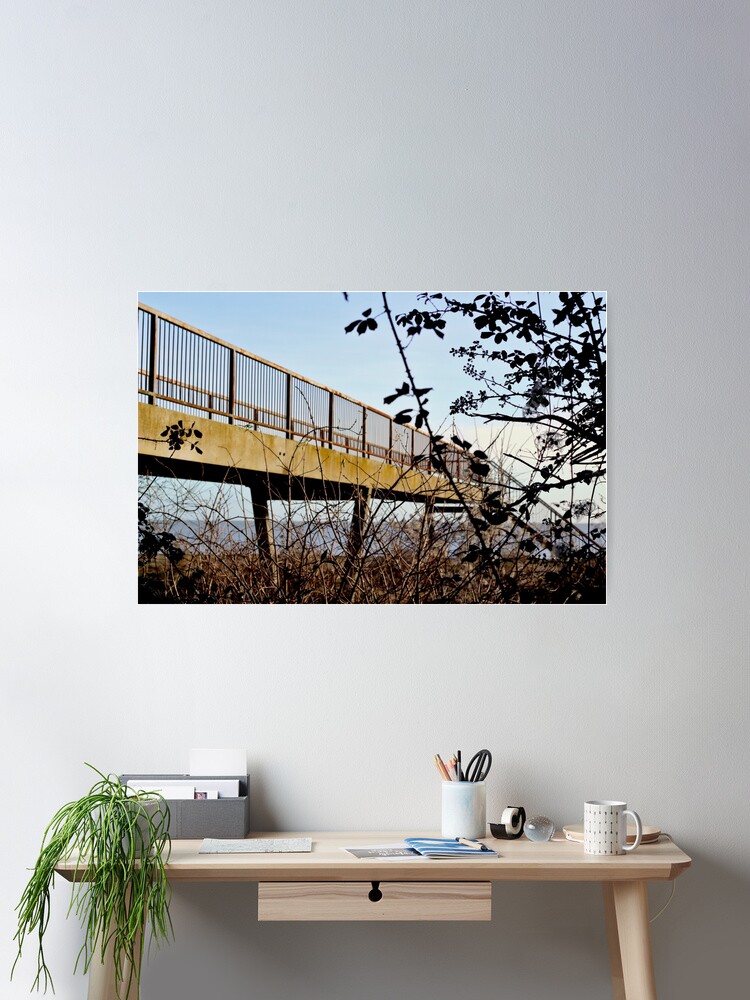This indoor photograph captures a minimalist home office setup, characterized by its clean lines and organized space. The room features walls painted in varying shades of white and gray, creating a bright yet subtle background. Dominating the scene is a light-colored wooden desk with thin legs, positioned against the wall. Beneath the desk is a single sliding drawer.

On the left side of the desk, a vibrant green plant in a cup cascades over the edge, adding a touch of nature to the composition. Next to it is a gray container holding a couple of white envelopes, and in front are assorted papers, including a card and a booklet. A white mason jar filled with pens, pencils, and scissors sits next to a tape dispenser.

In the middle section of the desk lies a classic white coffee mug. Toward the right end of the desk, a small glass globe is placed next to a cylindrical desk lamp with an articulated arm, also in white. Mounted on the wall above the desk is an artful photograph depicting a concrete walkway bordered by a black metal fence. The walkway image includes silhouettes of trees, completing the serene and tasteful aesthetic of this home office.